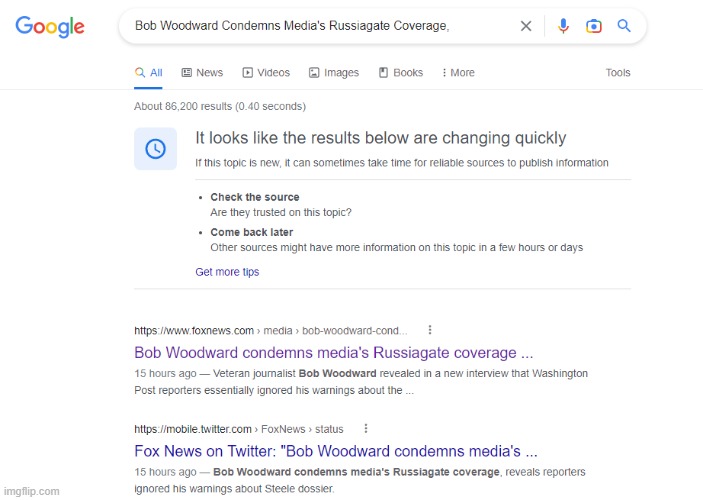The image is a detailed screenshot of a Google search results page. Positioned in the upper left-hand corner is the recognizable Google logo, followed by a search bar containing the query: "Bob Woodward condemns media's Russiagate coverage." Directly below the search bar, there is a row of Google search categories: All, News, Videos, Images, Books, and More. On the far right of this row is an option labeled Tools.

Beneath these categories, an informational section indicates that there are approximately 86,200 results for this search. The section also suggests that reliable sources may take time to publish information if the topic is new and advises users to check the credibility of sources, highlighting that additional details might emerge over the following hours or days.

Below this advisory, the top search result originates from Fox News. It features the headline, "Bob Woodward condemns media's Russiagate coverage," and was posted 15 hours ago. The second result is from Twitter, specifically Fox News' Twitter profile, with a similar headline truncated to: "Bob Woodward condemns media's..." This tweet was also posted 15 hours ago. Notably, the bottom left corner of the screenshot has a watermark from imgflip.com.